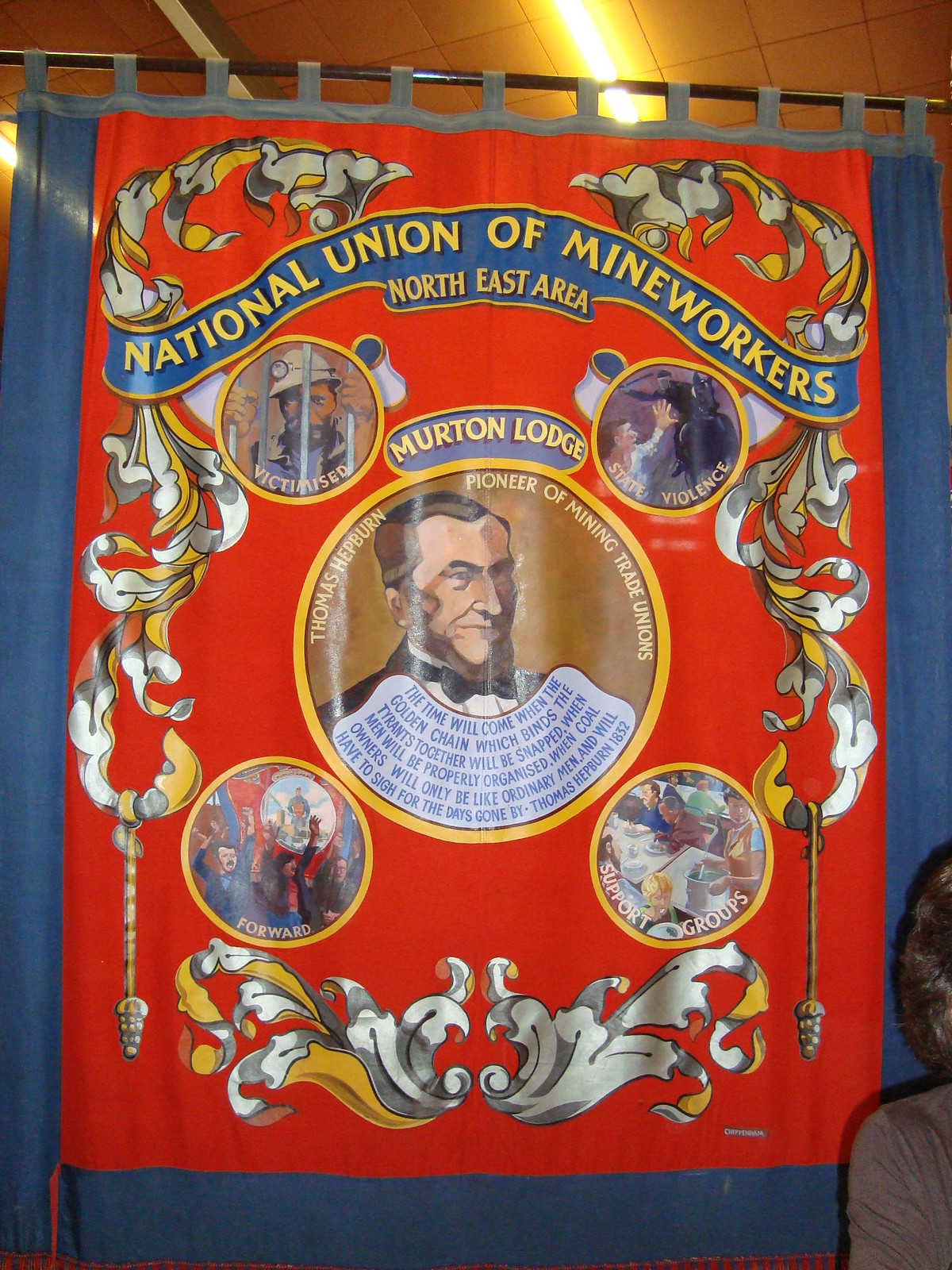This photograph captures a vibrant, red banner adorned with ornate floral and scroll patterns in silver and gold. Suspended from a rod against a blue curtain, the banner prominently features a blue ribbon near the top with the yellow text "National Union of Mine Workers Northeast Area." Dominated by a central circle, the banner depicts a caricature of Thomas Hepburn, identified as the "pioneer of mining trade unions," with the associated text "Merton Lodge" above him. Surrounding this central image are smaller illustrated vignettes, including a man behind bars labeled "victimized," and another scene showing state violence, where a mounted man wields a stick at another figure with raised hands. Further text on the banner provides a historical quote from Thomas Hepburn dating back to 1832, speaking of a future where the oppressive "golden chain" binding tyrants will be broken. The banner's rich hues and traditional design elements juxtapose its modern vibrancy, creating an appearance reminiscent of historic union banners.